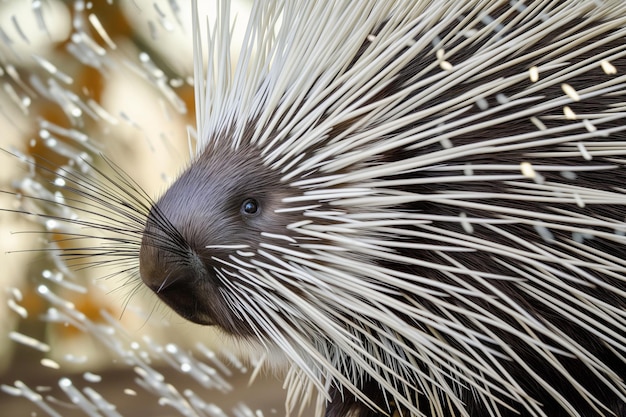This detailed color photograph captures a strikingly close-up view of a porcupine's face. The primary focus is on the intricate features of the porcupine, prominently showcasing its large black eye and long, dark black whiskers extending from its snout. Each quill is clearly visible due to the magnification, revealing a stark contrast between the quills’ pure white coloration and the porcupine's underlying dark fur, which ranges from brown to nearly black. The quills start around the porcupine’s nose and eyes, continuing to cover its head and trail down its back. The background is blurry, creating an illusion that some of the white quills might be floating or shooting out, though this effect could be attributed to the abstract design in the backdrop rather than actual motion. Overall, the image provides an intimate and detailed study of the porcupine, with an emphasis on its facial features and quills against a less distinct, blurred background.